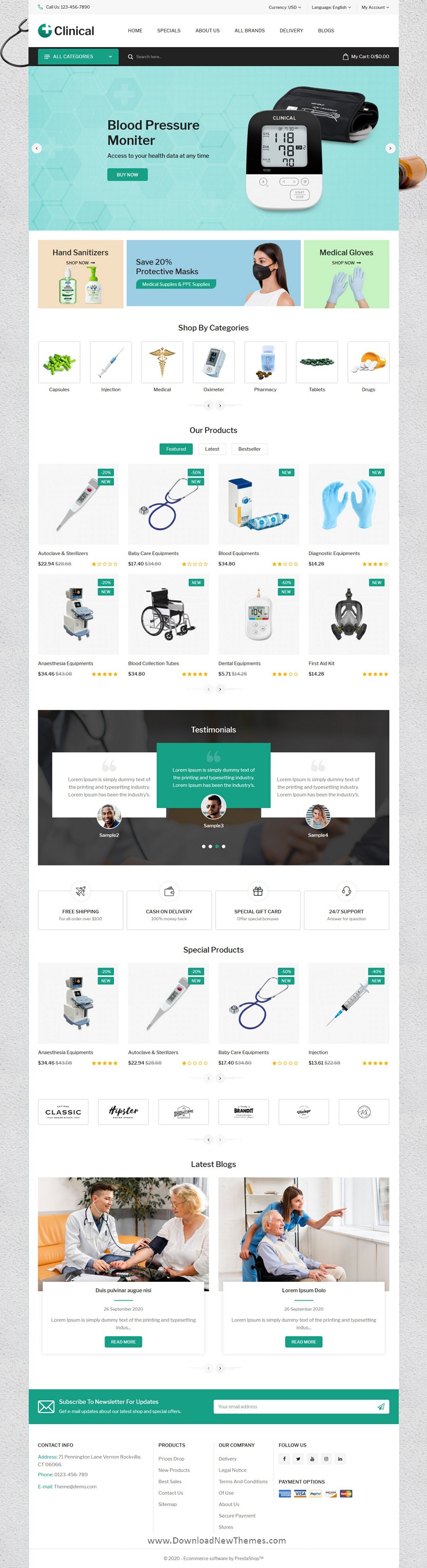The website "Clinical" is prominently displayed in the upper left corner of the page, followed by a contact number "1-234-567-890". To the right of the "Clinical" logo, the navigation menu includes links to "Home," "Specials," "About Us," "All Brands," "Deliver," and "Blogs." Above this menu, users will find a strip containing options for choosing currency (default set to USD), language (default set to English), and an account drop-down menu labeled "My Account."

Below the primary menu, there is a black strip. On the left side, a green drop-down menu labeled "All Categories" is displayed with white text. Next to it, a search bar with an accompanying search icon is situated, and on the far right, a cart icon with the label "My Cart" indicating a current total of "$0.00" is visible.

The section below features a light green background banner advertising a "Blood Pressure Monitor," which emphasizes accessibility to health data at any time. A green "Buy Now" button with white text is prominently displayed. To the right of this text is an image of a blood pressure monitor.

Beneath this banner are three rectangular advertisements arranged in a row. The left rectangle, set against an orange background, promotes "Hand Sanitizer" with a "Shop Now" directive and features images of two bottles of hand sanitizer. The center rectangle, on a blue background, offers a "Save 20%" deal on "Protective Masks, Medical Supplies, and PPE," with the text "PPE Supplies" highlighted.